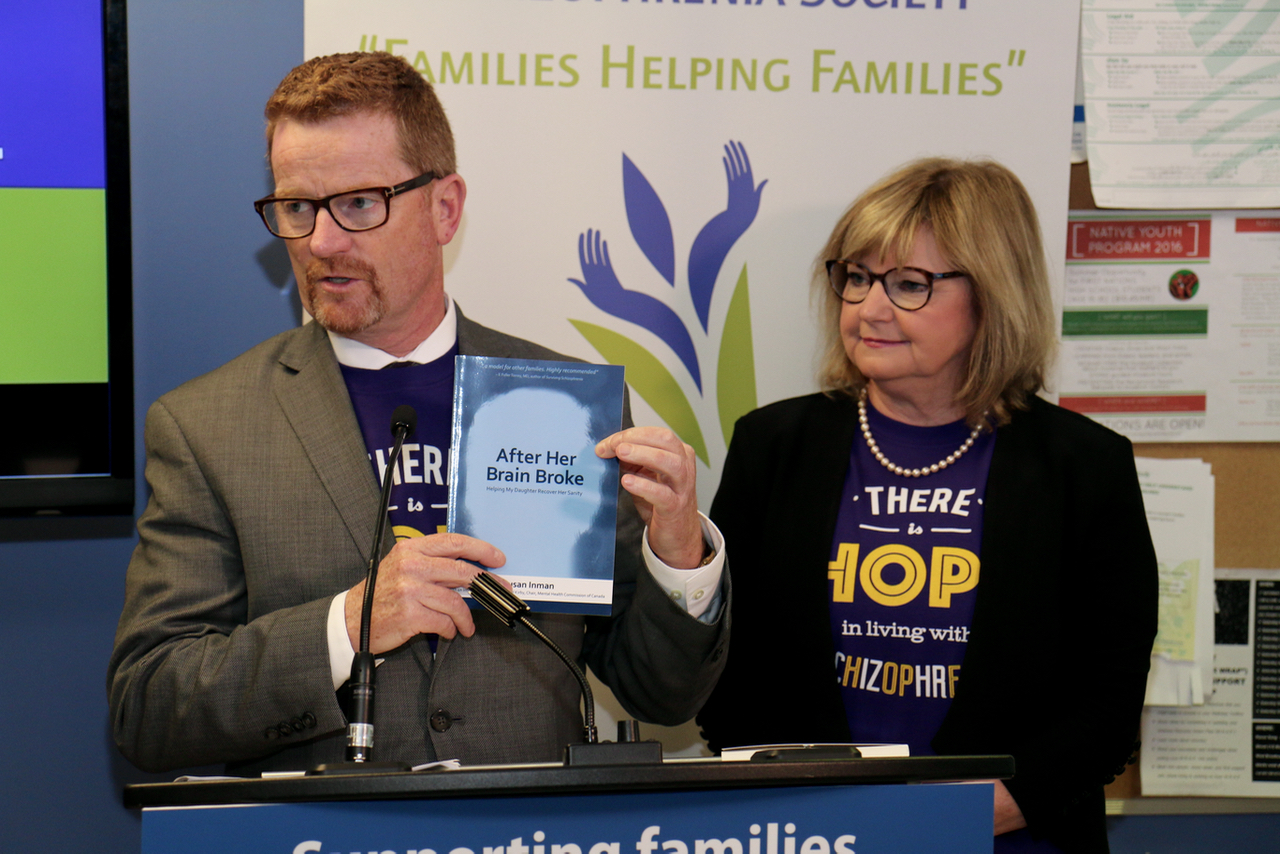This image captures a detailed scene at an event promoting mental health awareness. In the background, a white poster reads "Families Helping Families" in green lettering, accompanied by artistic designs resembling hands and decorative corn borders. At the forefront, a man with short red hair, a goatee, and black-framed glasses stands at a podium. He is holding a book titled "After Her Brain Broke" by an author with the last name Inman. The man is dressed in a gray suit jacket over a blue shirt with a white collar, and he speaks into a microphone as he faces slightly to the left. Beside him stands a woman wearing a black suit jacket over a blue T-shirt that partially reads, "There is Hope in Living with Schizophrenia." She also wears glasses and a pearl necklace. Both individuals are addressing the audience with a shared focus on supporting families dealing with mental health challenges, as highlighted by the podium's inscription, "Supporting Families."